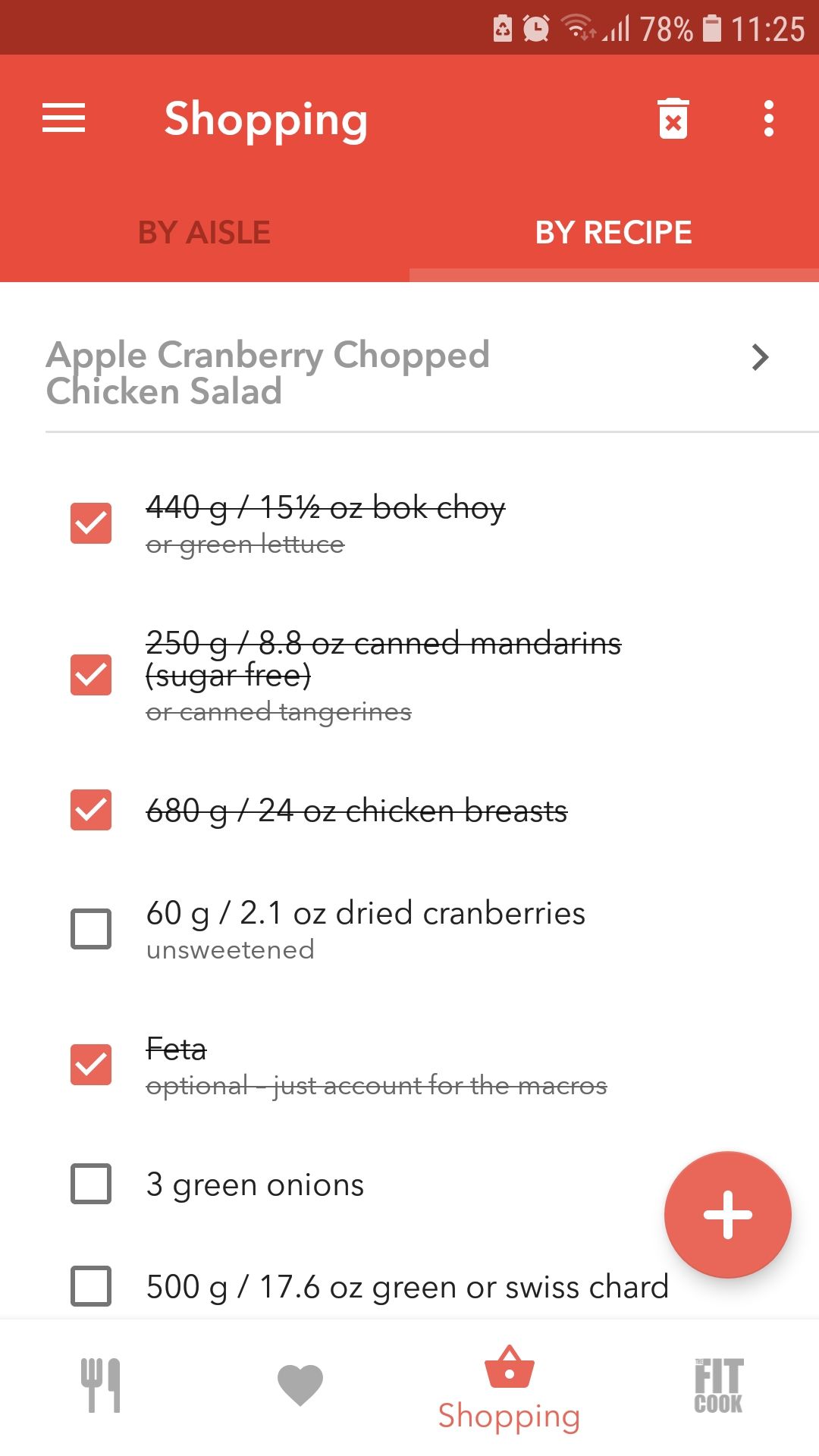This screenshot captures a mobile application interface showcasing a grocery shopping list. 

Starting at the top, a bold red bar spans the width of the screen. Within this bar, on the upper left corner, a white "List" button is prominently visible. Centered within this red bar, the word "Shopping" is displayed in bold white letters. Toward the upper right corner, there is a trash icon symbol with an 'X' on it, alongside a vertical ellipsis button (three vertical dots) for additional options.

Directly below the red bar, a tab navigation menu is displayed. The first tab says "By Aisle," while the second tab, "By Recipe," is currently selected and highlighted in bright white.

The main content area of the screen features a white background, where "Apple Cranberry Chopped Chicken Salad" is listed as the recipe title. Below the title, there are several checkboxes aligned with various ingredients for the cranberry salad. Some ingredients have been marked as acquired and are checked off, highlighted with a red box containing a white checkmark, while others are left blank with an empty white box indicating they have yet to be collected.